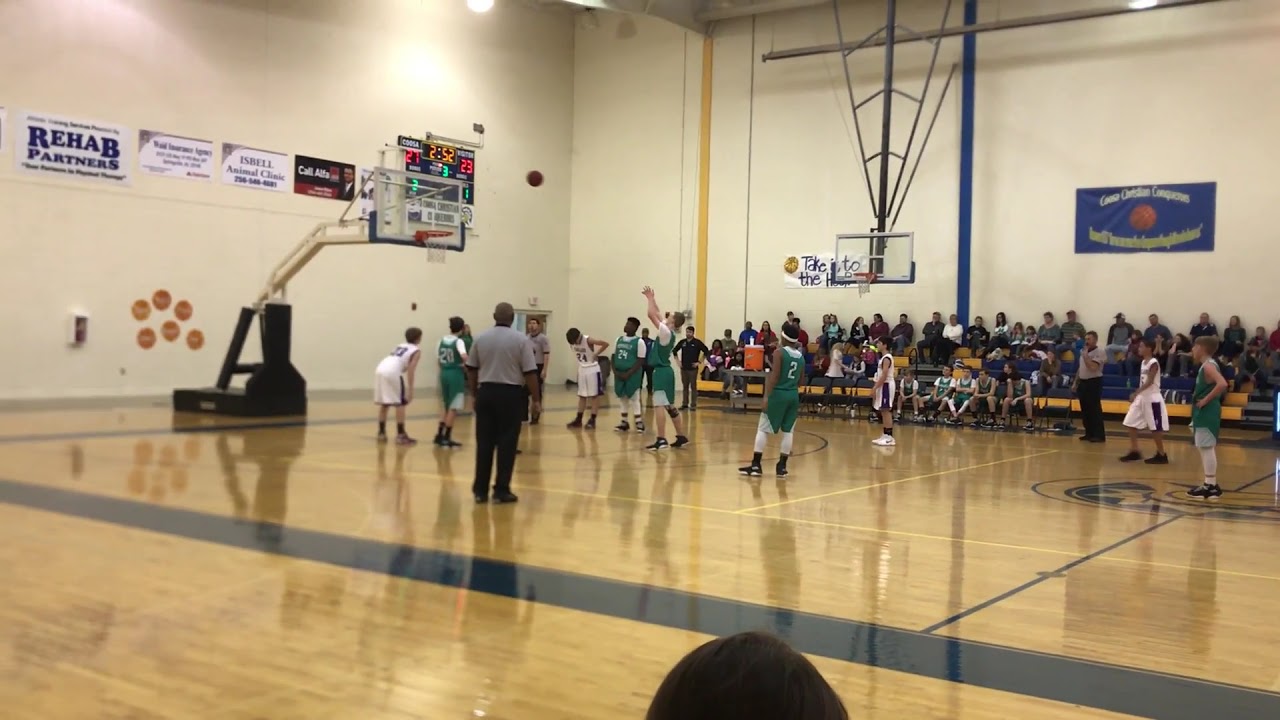This detailed snapshot captures an indoor basketball game inside a high-ceiling gymnasium with white walls and a shiny, tan-colored floor marked with court lines. The focal point is on the left side of the court, where children in green and white jerseys are actively playing. A player in green, with the number 2 on his uniform, is seen aiming a shot while others are positioned for a foul throw. To the left of this action, a digital scoreboard displays a tight score of 27-28 with 2 minutes and 52 seconds remaining in the game. Behind the scoreboard, numerous rectangular advertisements and a distinctive backdrop featuring rehab partners and basketball-themed shapes adorn the white wall. A fire extinguisher is also visible there. Spectators are sparsely seated in bleachers on the right, observing the game from behind another basketball net at half-court. Two referees are present, one near the players with his back to the camera, and another on the opposite side. The scene is completed with various banners and posters, including a prominent blue one with a basketball image in the middle, contributing to the vibrant ambiance of the gym.